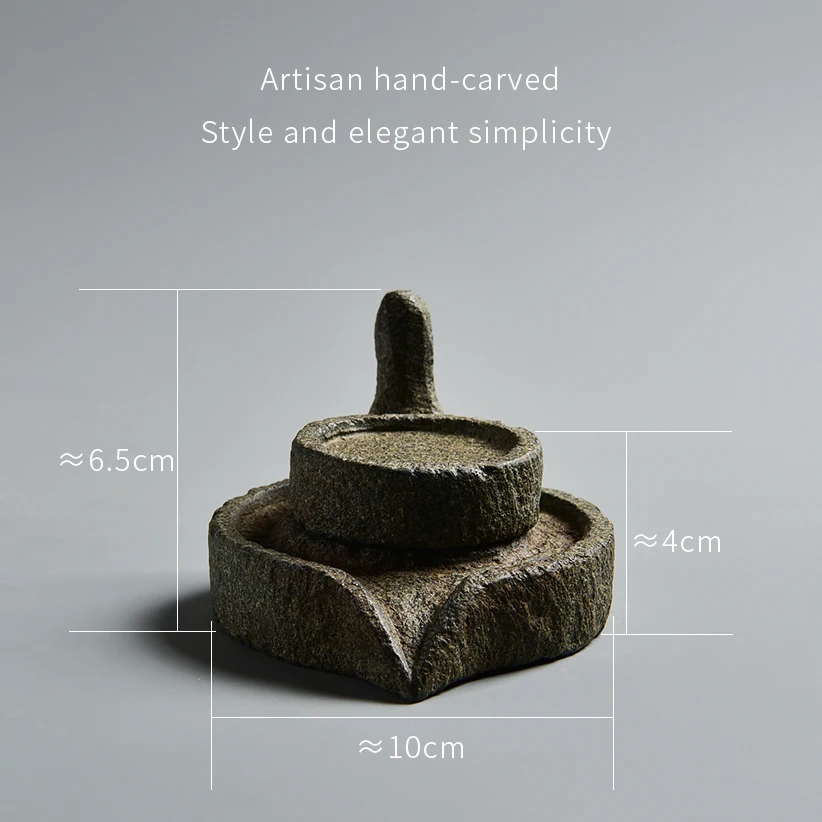The photograph showcases an artisan hand-carved stone object, epitomizing elegant simplicity. The structure consists of two cylindrical shapes, one stacked atop the other, with the larger serving as the base. The bottom cylinder, reminiscent of an ashtray, features a V-shaped notch at the front where side supports are separated. The top cylinder, smaller and ringed by a subtle lip, resembles a coaster. A long, handle-like stump extends from the back, making the object easy to grasp. The stone artifact, dark gray in color, includes a divot or spout designed for pouring. The image is overlaid with white text reading "Artisan hand-carved style and elegant simplicity." Dimensions are provided with lines indicating the measurements: 6.5 centimeters in height, 10 centimeters in diameter, and 4 centimeters in width. The backdrop of the image is a light gray.